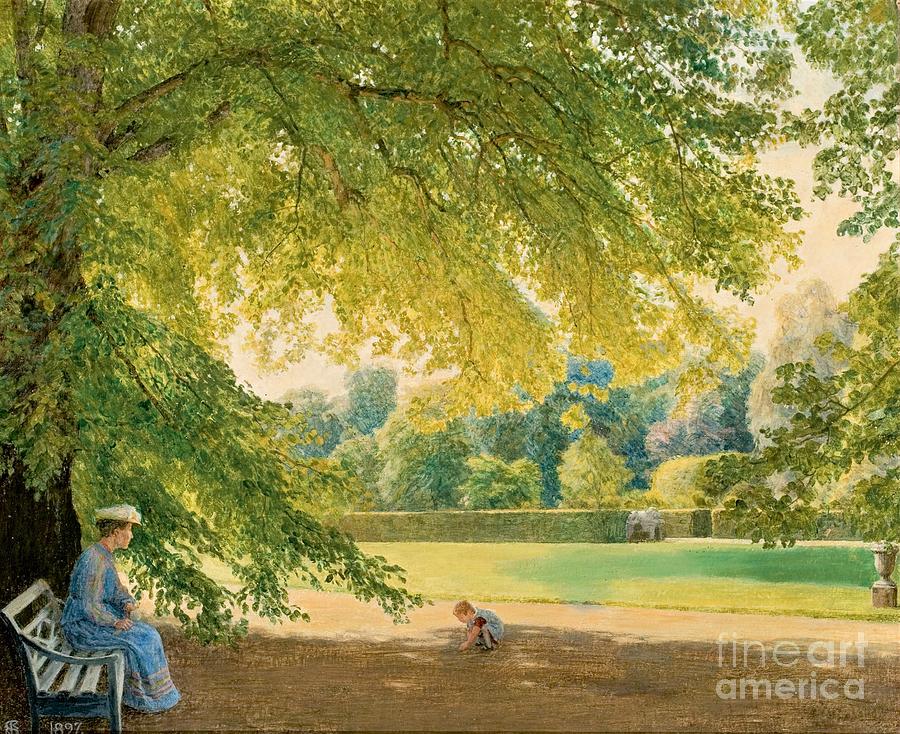This painting, possibly an oil painting dated 1897 and watermarked by Fine Art America, depicts a tranquil park scene from the 1800s. A woman, dressed in a long blue dress and wearing a hat, sits on a park bench to the left of the scene. She's intently watching her small, brown-haired son, who is crouched down and playing in the dirt. The boy appears to be pulling something from the ground under the shade of an enormous, leafy tree, which casts a vast shadow over both the mother and child. The background features a beautifully rendered landscape with a mix of green and yellow hues, hinting at varying types of foliage, including hedges and numerous trees. There's also a lawn in the distance and possibly a wooden or stone wall at its far edge. The sky, tinged with brownish-gray tones, suggests an overcast day, adding depth to the serene and historical atmosphere of the park setting.